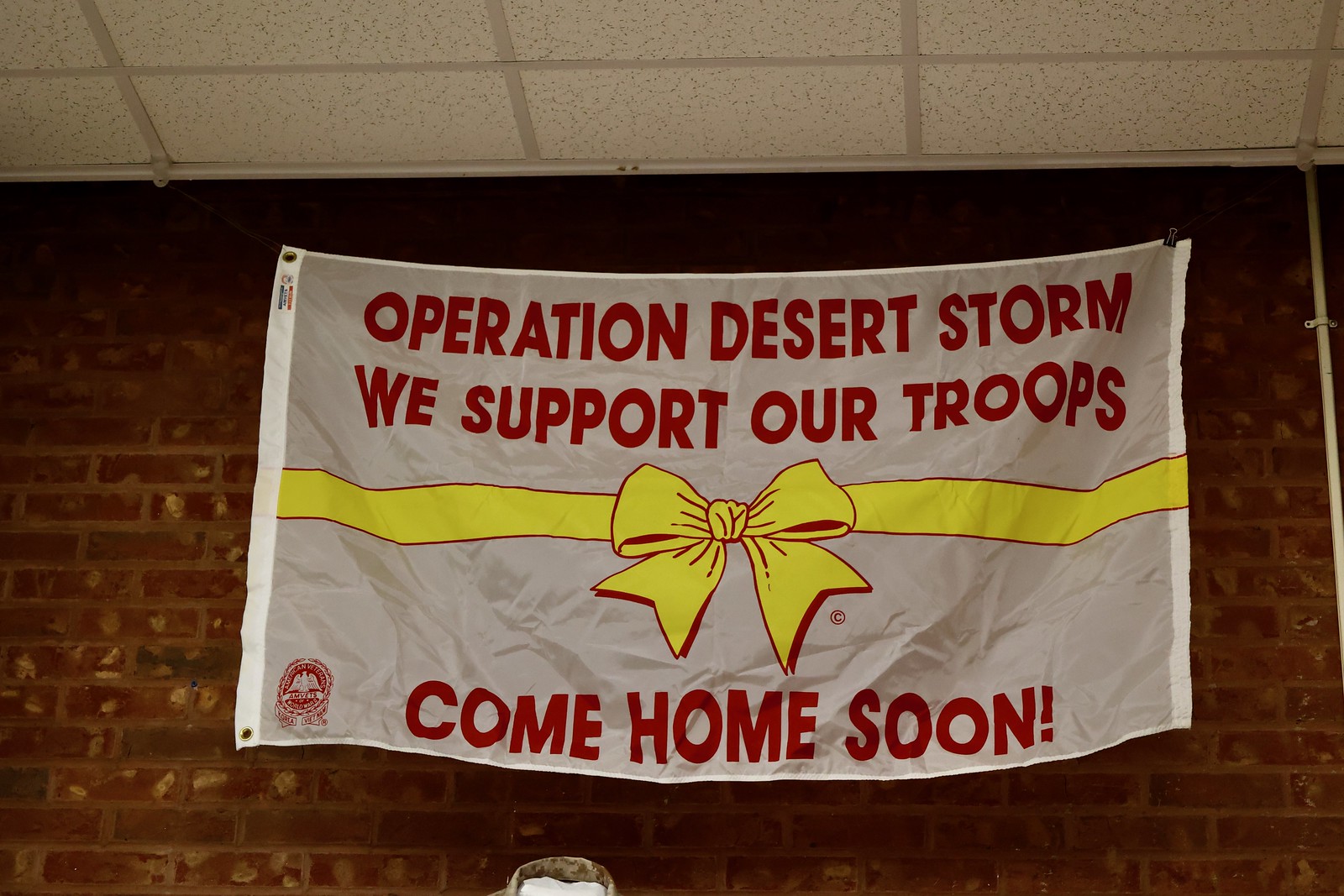The image shows an indoor scene with a banner hung against a dark red and maroon brick wall, beneath a ceiling of white tiles separated by light gray lines. The white fabric banner reads "Operation Desert Storm, We Support Our Troops, Come Home Soon" in bold, all-capital red sans-serif font, with text positioned both at the top and bottom. A prominent yellow ribbon, adorned with a thin red outline, is displayed across the center of the banner, tied in the middle to form the classic ribbon shape. The fabric of the banner shows noticeable wrinkles, suggesting it is made from a soft material. The banner is likely secured to the ceiling by a thin wire, as no visible fastenings can be seen. The image bottom hints at what appears to be the top of someone's head, reinforcing the indoor setting, which might be a venue for a support group for war veterans.